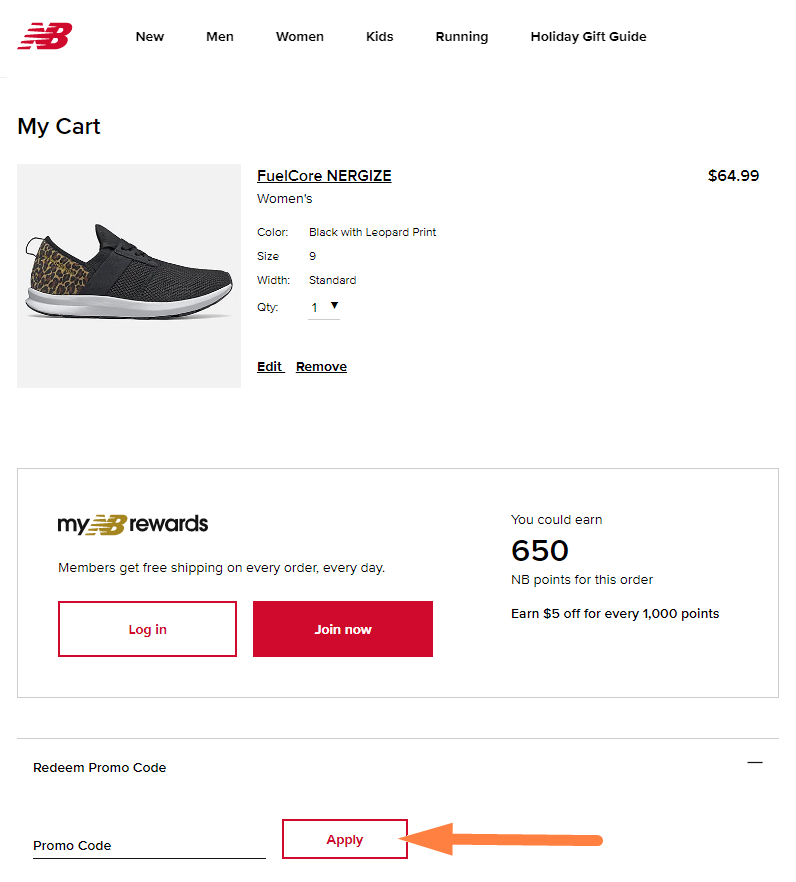This detailed screenshot from the New Balance website captures the "My Cart" page. In the upper left-hand corner, the iconic red "NB" logo, standing for New Balance, is prominently displayed. Adjacent to the logo, the top navigation menu features several sections including "New," "Men," "Women," "Kids," "Running," and a "Holiday Gift Guide."

Centered on the page is the shopping cart summary. Here, a women's pair of "FuelCore Nergize" shoes is listed. The shoes are primarily dark gray with a striking leopard print on the back. They feature a thick white rubber sole, combining both style and functionality. The shoes are priced at $64.99, in size 9 with a standard width, and the quantity selected is one. Options to "Edit" or "Remove" the item are provided for easy adjustments to the cart contents.

Beneath the cart summary, a banner ad promotes the "My Envy Rewards" program, highlighting that members receive free shipping on every order, every day. Two buttons are available: "Log In" for existing members and "Join Now" for new members. Additionally, a message indicates that this order could earn 650 Envy points, with a note that 1,000 points can be redeemed for $5 off.

At the bottom of the page, there is a section for applying promotional codes. A text box allows users to input their promo code, followed by an "Apply" button, which is specifically marked by an orange arrow for emphasis.